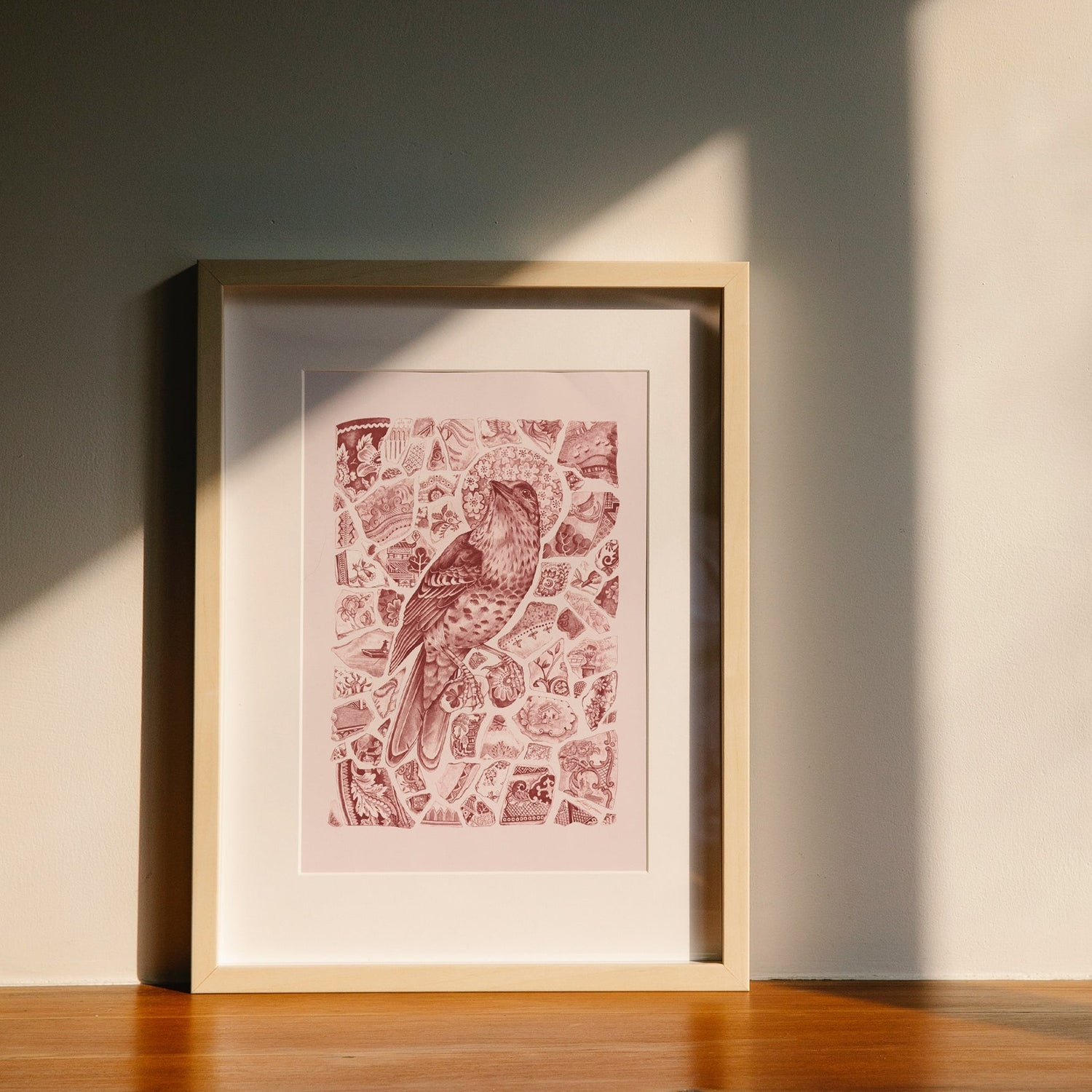The image depicts a light-colored wooden picture frame sitting on a light brown hardwood floor against a beige wall. Soft shadows indicate light filtering through a nearby window. The frame, with its subtle wooden texture, encases a white mat that accentuates the main artwork—an intricate digital illustration dominated by shades of dark red and white. The central figure in the illustration is a large bird, its belly adorned with spots, gazing upward. Surrounding its head is a ring of flowers, resembling a halo or a moon. The entire composition appears to be a collage, where numerous smaller elements merge to form the overarching image, creating an impression of complex, yet delicately dispersed patterns that include various indistinct shapes and designs.